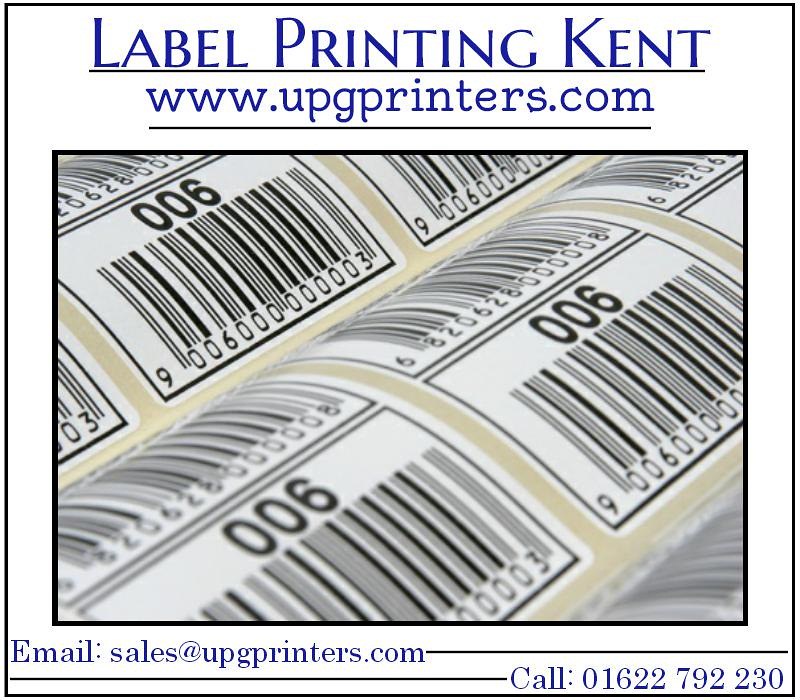The image appears to be a vintage digital advertisement for a label printing company based in Kent, featuring a minimalist and somewhat dated design. At the top of the image, set against a white background with black outlines, is the main heading in blue text: "Label Printing Kent." Below this heading, the website "www.upgprinters.com" is also displayed in blue and underlined with a black line. The central portion of the image showcases a prominent inset square outlined in black, containing a photo of multiple barcode stickers arrayed in neat rows, likely on a sticker sheet. Each barcode appears to have numbers above and below it, with repetitive sequences such as "006" and "900." At the very bottom of the image, again in blue text, is the contact email "sales@upgprinters.com," accompanied by another black line extending to the right. To the far right, near the bottom corner, the word "Call" is written in blue next to the phone number "01622 792 230." The overall design and content suggest it is an advertisement, possibly from an earlier digital era, for a company specializing in barcode labels and related printing services.